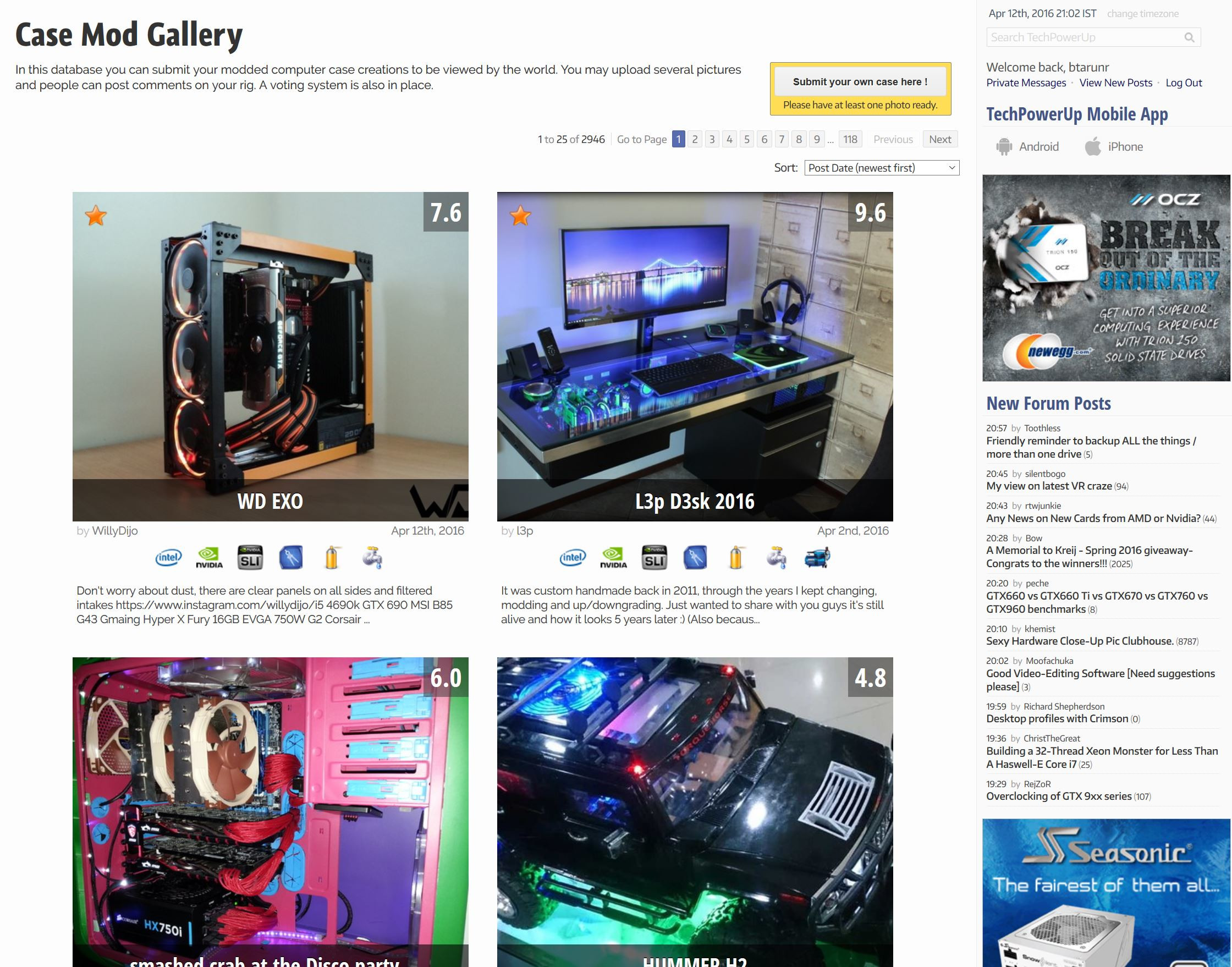In the image, we see a screenshot of a web page titled "Case Mod Gallery," which is displayed prominently in black letters in the upper left corner. Below the title, there is fine print that reads: "In this database, you can submit your modded computer case creations to be viewed by the world. You may upload several pictures and people can post comments on your rig. A rating system is also in place." To the right of this text, there is a button outlined in yellow that says "Submit Your Case Here."

Below this information, the page indicates that there are 7,946 case mods displayed across 118 pages, and users can select which page to navigate to. On the current page, there are four showcased cases:

1. The first case, located in the top left, is labeled "W-D-E-X-O" and features a rating of 7.6. The case appears to integrate three speakers on its left side, with intricate internals visible. Inside, several black and red wires are connected to a central device, possibly a circuit board.

2. In the first row, second column, the case is labeled "L-P-3-D-3-S-K-2-1-2-0-1-6-2016." This setup resembles a computer desk, complete with a monitor displaying a twilight image of a bridge illuminated by white lights reflected in a body of water. The desk has a glass top, which reflects the monitor's image, and is equipped with a keyboard, speakers, a touchpad, and headphones on a stand. Beneath the desk, there are drawers on both sides, with additional filing cabinets seen in the background.

3. The third case, located in the second row, first column, is intriguingly named "Smashed Crab at the Disco Party." The interior showcases circuit boards, a hard drive, and numerous red cables connecting various components, including the motherboard. The case’s color scheme is vibrant, with pink internals, light blue plug attachments, and a purple device in the bottom right corner.

4. The fourth case in the bottom right resembles a Jeep, complete with large studded wheels and a black body. However, the interior reveals it to be a functional computer. This unique mod has a rating of 4.8.

Overall, the "Case Mod Gallery" web page provides a detailed platform for users to display their custom computer case designs, complete with images, descriptions, and user interactions through comments and ratings.